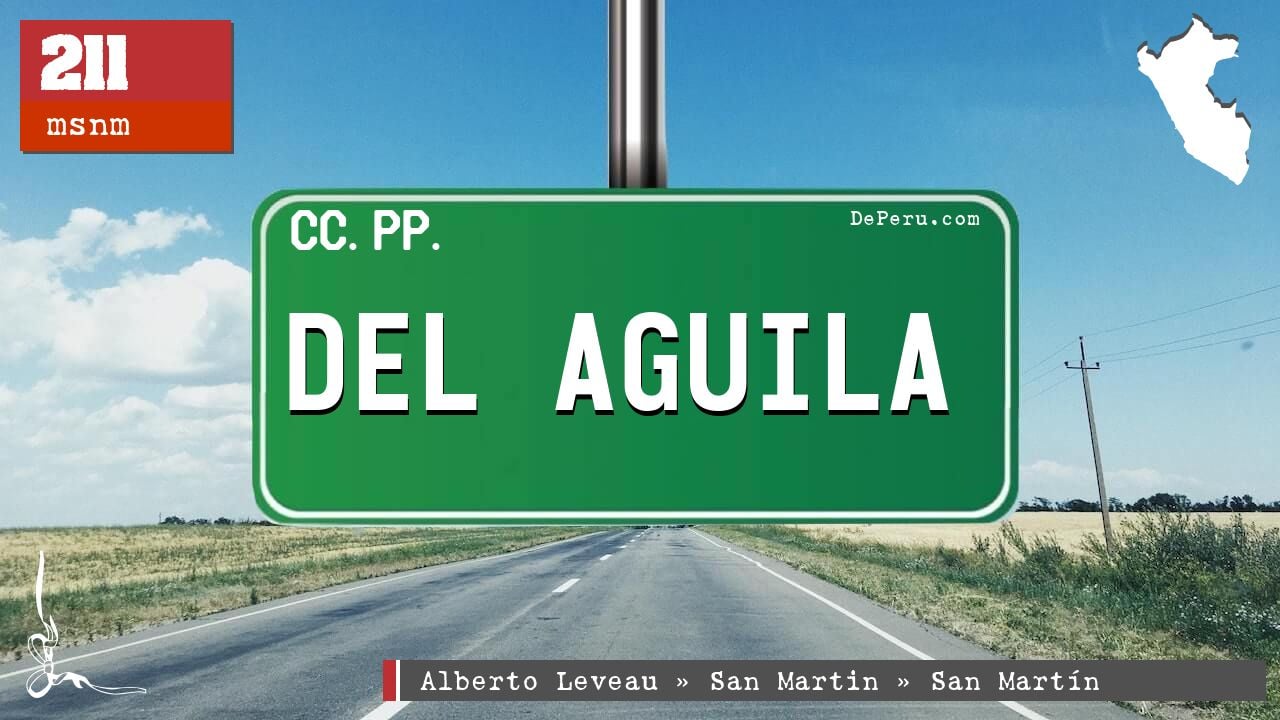The image depicts a country scene of a two-lane paved highway stretching into the distance, flanked by farmland on both sides. Power lines run along the right side of the road, with some bushes nearby, creating an open and expansive ambiance. The sky above is a vivid blue, adorned with scattered white clouds, occupying the majority of the background.

Prominently positioned in the middle of the image is a large green license plate bearing the inscription "DELAGUILA" in bold white letters. In the upper left corner of the license plate is the acronym "CCPP," while the upper right corner reads "deperu.com." This likely indicates a connection to Peru. Further enhancing the local flavor, the bottom of the image displays the text "Alberto Laveau San Martin," suggestive of the region or the photographer's name.

In the upper left corner of the image, a red box with the white numeral "211" and the acronym "MSNM" below it can be seen. This suggests elevation in meters above sea level. The upper right corner likely features an outline of Peru in white, though it's somewhat unclear.

Adding to the surreal and layered nature of the scene, a metal bar descends from the top of the image, evoking the impression that the photo might be taken from inside a vehicle, possibly giving a sense of a road trip scenario. The composition brings a concentrated focus on the details upfront, creating a vibrant tapestry of colors with green, blue, and black dominating the palette.